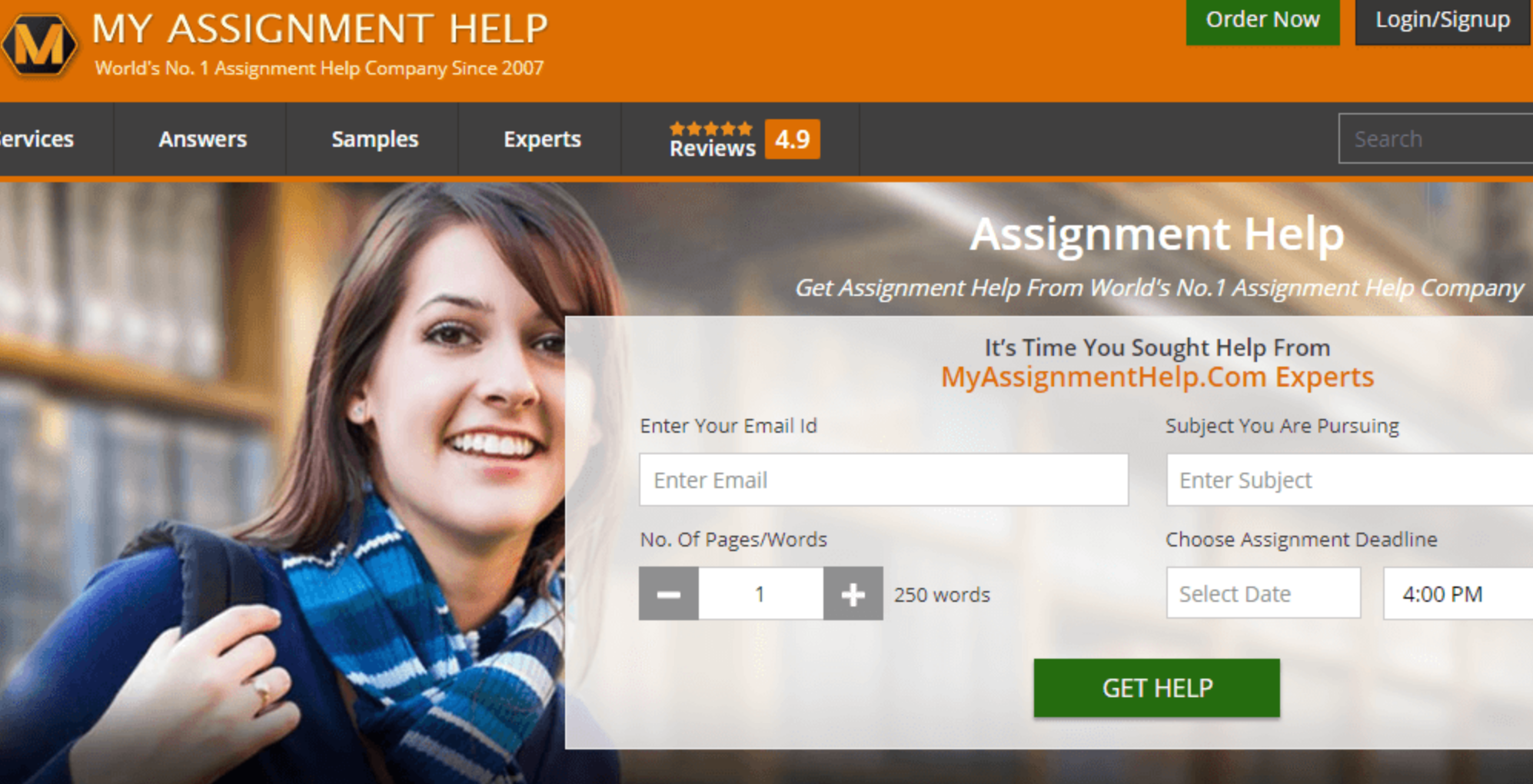The image features a top banner in orange with a capital letter 'M' in the center. The background is black, and the 'M' is also orange, surrounded by the text "My Assignment Help" in white print. Beneath this, it reads, "World's Number One Assignment Help Company since 2007," with "Number One" presented as "No. 1."

To the right side of the banner, there's a green "Order Now" button with white text. Adjacent to it, on a black background, the text "Login / Sign Up" appears in white.

Lower on the page, a charcoal banner displays the sections "Services," "Answers," "Samples," "Experts," and "Reviews," with a rating of "4.9" enclosed in an orange box.

Further down, a graphic depicts a woman wearing a blue scarf, blue shirt, and a navy blue backpack. She has a ring on her ring finger. The text to the side reads, "Assignment Help: Get Assignment Help from World's Number One Assignment Help Company."

Below this, a box prompts users with: "It’s time you sought help from MyAssignmentHelp.com Experts." It requests details such as email ID, the subject being pursued, the number of pages/words, and the assignment deadline. This is followed by a green banner with the text "Get Help" in white print.